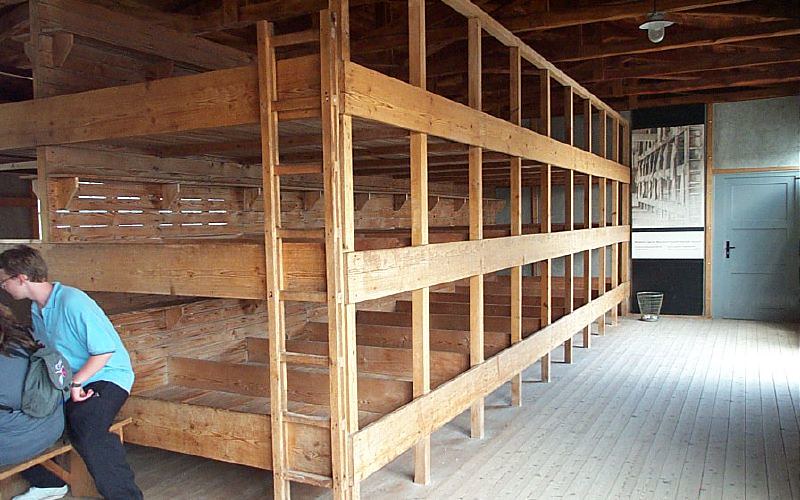The color photograph depicts the interior of a rustic cabin, likely part of a sleepaway camp. The space features plank wood floors and exposed wooden beams above. Dominating the room is a massive, hand-built three-tier bunk bed system, each tier comprising eight wooden bunks. The bunks, constructed with simple wood and lacking mattresses, have dividers between them to prevent occupants from rolling over to the neighboring bed. 

In the bottom left corner, a teenager with brown hair, wearing an aqua-colored t-shirt, dark pants, glasses, and a wristwatch, is partially visible. He is squatting near a bench where a gray duffel bag or a sleeping bag rests. The cabin features a screen door and a standard green door at the far end, leading to another wooden structure visible in the background. The ceiling has a rudimentary light fixture hanging from the beams, and a wire wastebasket can be seen near the doors. The entire scene, stark and unadorned, evokes a stark and utilitarian atmosphere characteristic of communal living spaces at camps.